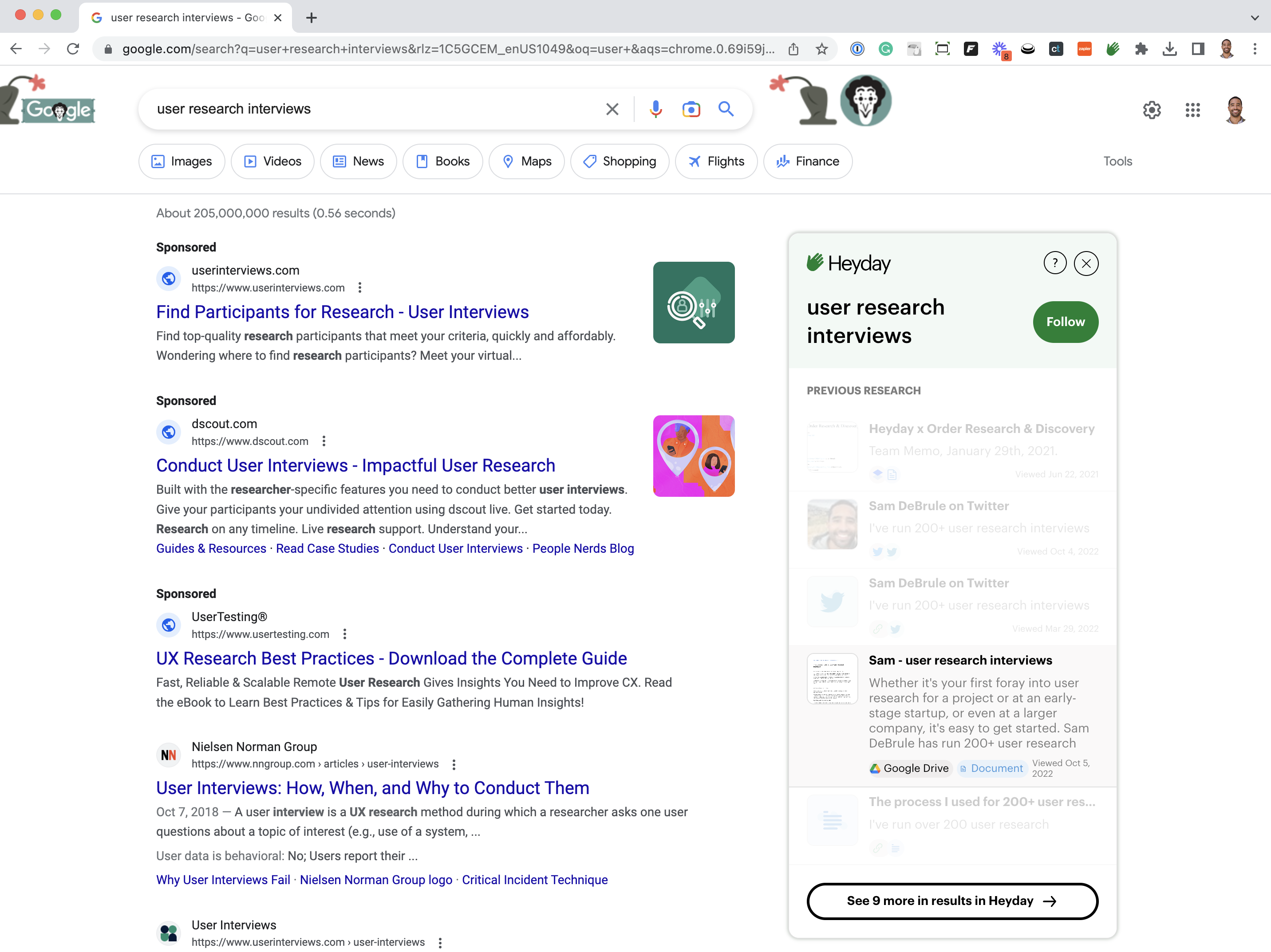The screenshot captures a Google search results page for the query "user research interviews." The interface is framed by a light grey header bar that reads "User Research Interviews" on the browser tab. Below the header, an address bar sits with various icons. The main search box features the iconic Google logo on the left and several functional icons on the right.

Directly under the address bar are navigation links labeled: Images, Videos, News, Books, Maps, Shopping, Flights, and Finance. 

The search results area displays four visible results on the left-hand side of the page. The first three entries are identified as sponsored results, highlighted by larger blue fonts. These include:

1. "Find Participants for Research User Interviews"
2. "Conduct User Interviews"
3. "Impactful User Research"

Additionally, there are smaller subtexts like "UX Research Best Practices," "Download the Complete Guide," and "User Interviews: How, When & Why to Conduct Them."

To the right of these listings, there’s a semi-transparent button that says "Heyday: User Research Interviews." The button includes a "Follow" option. At the bottom of the results column, a link prompts users to “See nine more results in Heyday.”

The entire screenshot lacks a distinctive border on the left, right, and bottom edges, giving it an open layout appearance.